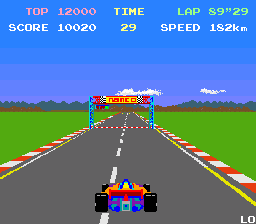The image is a small, square screenshot from an old Nintendo video game, likely an F1 racing game developed by Namco. Dominating the center of the pixelated and vibrant scene is a low-to-the-ground race car, colored in shades of orange, blue, purple, and red, with the driver's helmet visible due to the open-top design. The car is positioned over the dotted white line in the center of a two-lane road, which stretches into the distance, leading to a visible finish line marked with the name "Namco." On either side of the road are yellow lines, followed by red and white stripes, green grass, and a bright blue sky overhead. The game's user interface displays various stats: "top 12,000," "time lap 89.29," "score 10,020," and "speed 182 km." Some text also appears at the bottom right corner of the screen, showing "low" spelled out as "L-O." The image evokes a nostalgic feel with its vintage, colorful, and highly pixelated graphics.